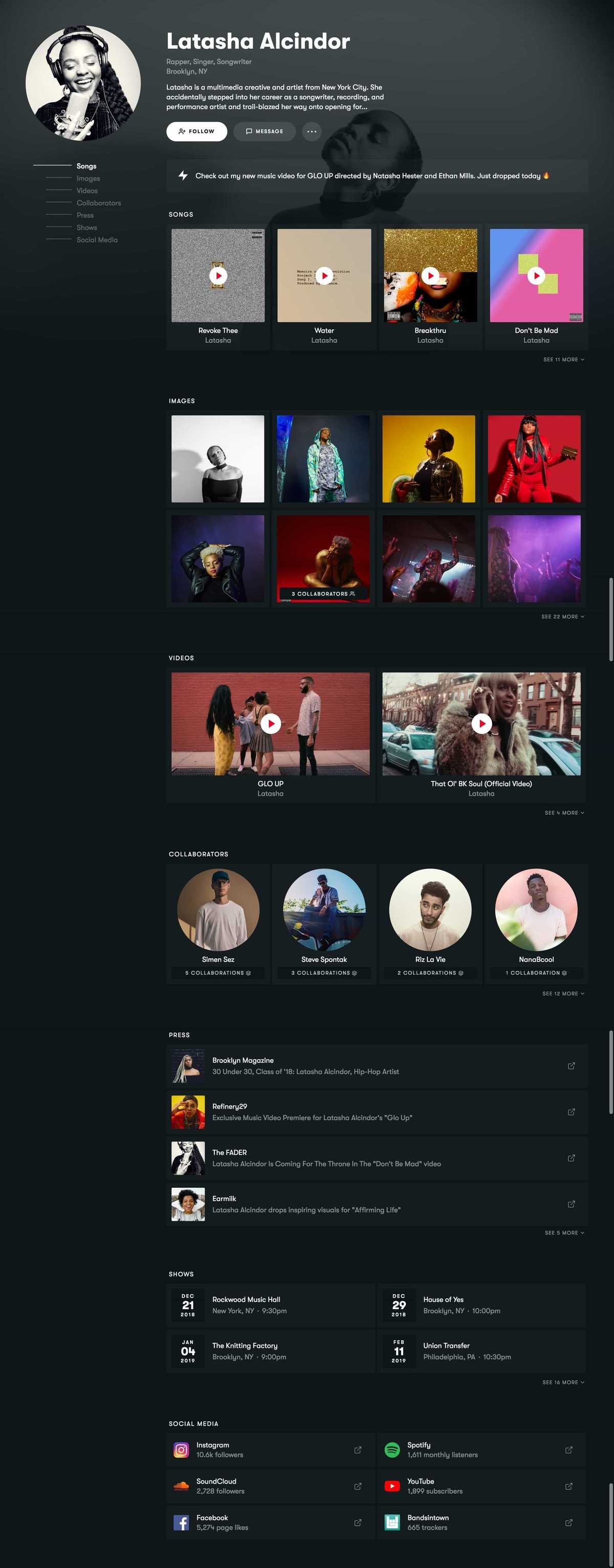The screenshot displays a detailed music page dedicated to Latasha Alcindor, a multifaceted artist from Brooklyn, New York. The top section features her name prominently, along with options to follow her. Latasha is described as a rapper, singer, songwriter, and multimedia creative with a strong foothold in the music industry as a recording and performance artist, and trailblazer.

The page showcases a collection of her songs, including "Revoke 3," "Water," "Work Through," and "Don't Be Mad," with play options available for each track.

Below the song list are eight distinct images of Latasha, each set against different colored backgrounds—white, black, yellow, and red—highlighting her versatility and eclectic visual style.

Further down, two of her music videos are displayed, offering a glimpse into her dynamic performance capabilities.

Towards the bottom, the webpage lists four collaborators, indicating individuals or groups she has worked with. Accompanying this is a press section that features articles and interviews about Latasha, along with dates for her upcoming shows.

The page also includes links to her social media profiles and where her music can be streamed. The entire page is set against a stylish black background, providing a sleek and modern aesthetic.